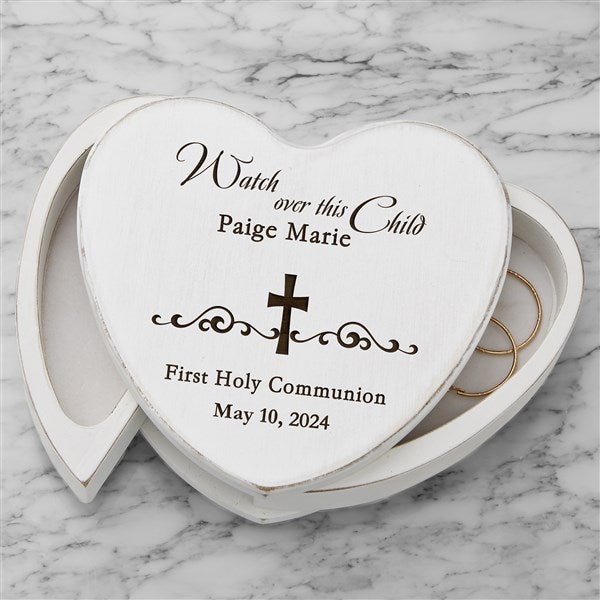This color photograph captures a heart-shaped, white ceramic jewelry box resting on a striated black, white, and gray marble countertop. The jewelry box bears the inscription, "Watch over this child, Paige Marie, 1st Holy Communion, May 10th, 2024," written in black lettering. Central to the inscription is a black crucifix with decorative curly cues emanating from either side, symbolizing Paige Marie's First Holy Communion. The box features a hidden compartment that opens from the middle, revealing two gold hoop earrings in the right compartment, while the left compartment remains empty. The edges of the ceramic box are slightly darkened, adding a touch of vintage charm to the piece.